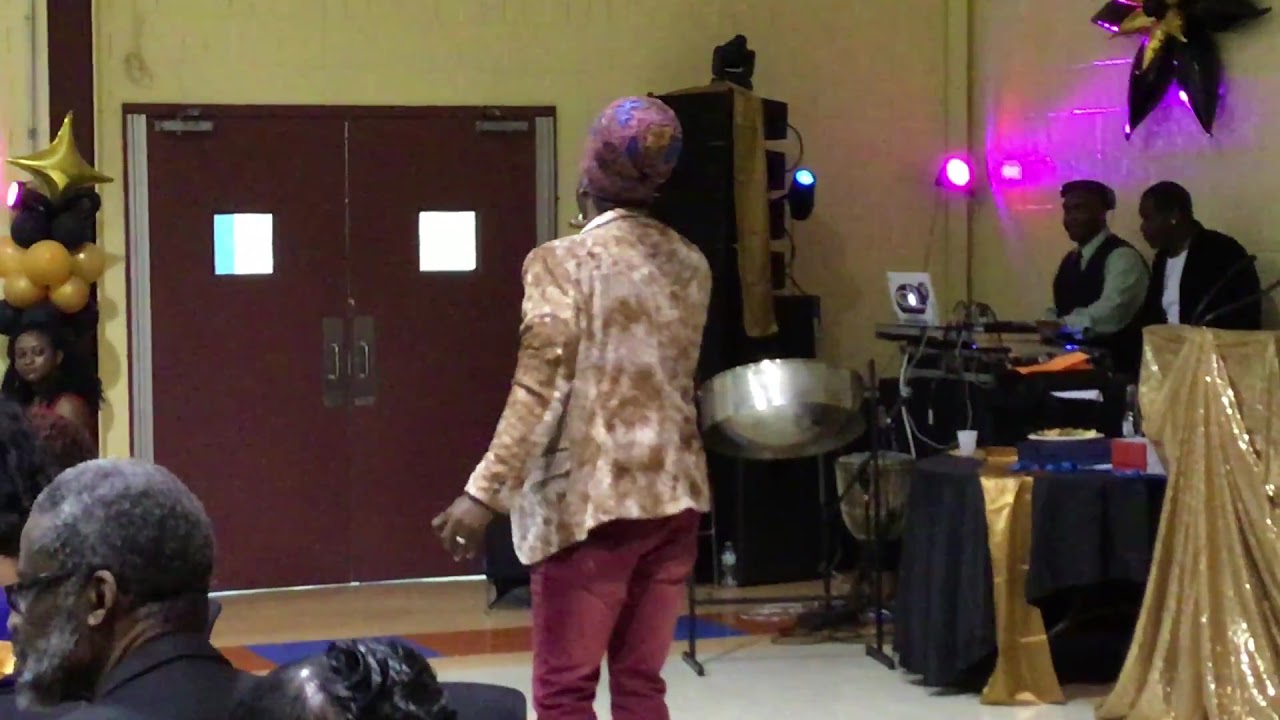The photograph captures an indoor African-American gathering, possibly a party or a church event, set in a multi-purpose room with yellowish-beige walls. Dominating the background of the image are a pair of dark red double doors with windows. On the right side, there's a DJ booth adorned with shiny gold and black fabric, housing DJ equipment and a laptop, flanked by two DJs. Nearby, another person stands adjacent to the booth. The back of a woman, clad in a fancy beige and white patterned jacket, purple pants, and a colorful purple-blue-yellow headdress, is prominently central in the photo, appearing to sing or address someone. To the left, a younger girl sits quietly, and an older male's profile is visible in the foreground. Decorations throughout the room include shiny stars, balloons, and a balloon sculpture on the left composed of gold, black, and yellow balloons, adding a festive touch to the space.